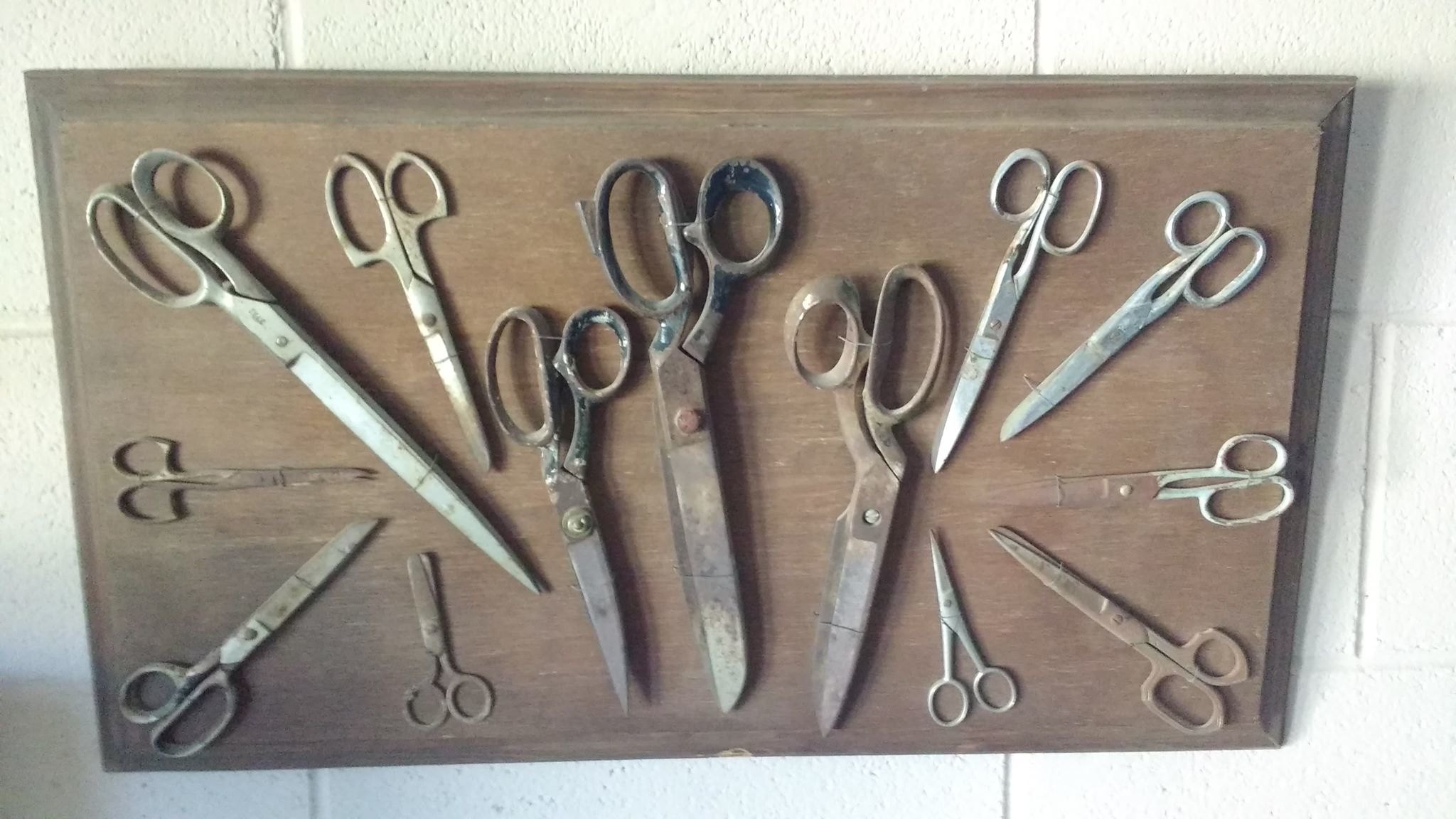A wooden plaque is mounted on a white-painted brick wall. The plaque, or possibly a cutting board, displays an array of scissors in varying sizes and conditions. The largest scissors are centrally positioned, while smaller pairs fan out towards the edges. The scissors are of different types, including large fabric shears and small, blunt child scissors. Some of them are rusted, exhibiting a brownish hue alongside the silver ones. The overall display combines a mix of old and new tools, creating an intriguing wall hanging that evokes a sense of a tool shed or a barber's collection.